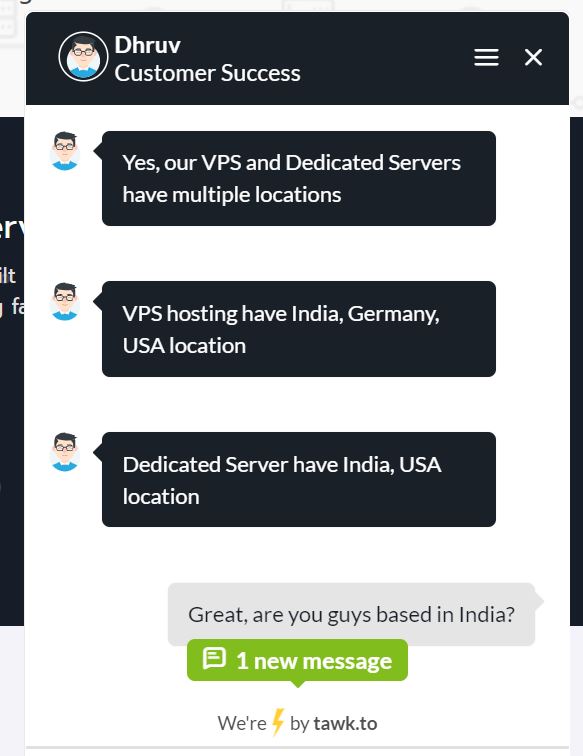In the upper left corner of the image, the name "DHRUV" is displayed prominently, with the words "Customer Success" directly below it. An avatar is shown nearby, featuring a person with a pale complexion, dark hair, glasses, and a blue shirt. The background for the upper portion of the image is black.

Adjacent to this section on the right, there is a menu icon and an "X" for closing, all set against a black background. The main content appears to be a messaging interface. The text conversation includes three main messages, each in white font on a black background:

1. "Yes, our VPS and dedicated servers have multiple locations."
2. "VPS hosting has India, Germany, and U.S. locations."
3. "Dedicated servers have India and U.S. locations."

To the right of these messages, another message appears in a gray background with black font that reads, "Great, are you guys based in India?"

Below this, a green pop-up with white font notifies, "One new message."

At the bottom, the phrase "We're by TWK.TO" is noted, where the words "we're" and "by" are separated by a lightning strike icon in yellow color.

The overall color scheme includes black, white, blue, light tan, gray, green, yellow, and white once again. A vertical black strip runs along the image's right edge, providing a balanced and organized visual structure.